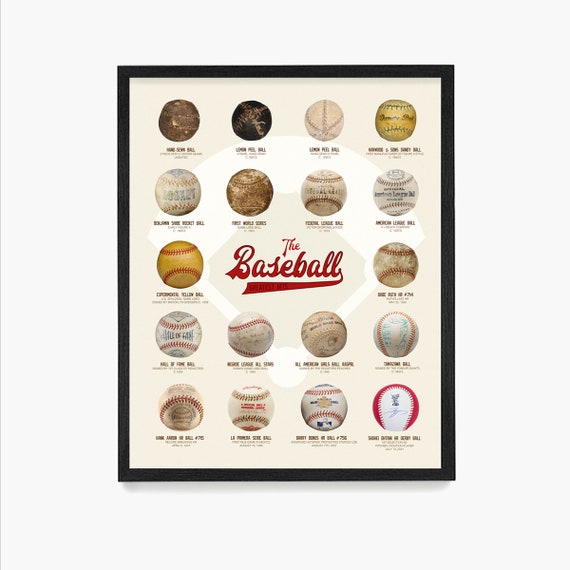This image features a chart showcasing the evolution of baseballs, encased in a black-framed art piece. In the center, the title "THE BASEBALL" appears in large, red cursive letters, underlined with a connecting line. Surrounding the title is a subtle silhouette of a baseball field, providing a nostalgic backdrop. Arranged in a four-column by five-row array, the chart displays 18 baseballs, starting from the top left with the oldest, brown and unrecognizable as a modern baseball, to the bottom right with a pristine white baseball, encircled by red stitching. Each ball represents a different era, detailing the changes in design and color, including white and yellow variations and ones with prominent lines. Small, unreadable writing beneath each ball suggests significant historical details, and many balls feature signatures that are too small to discern.